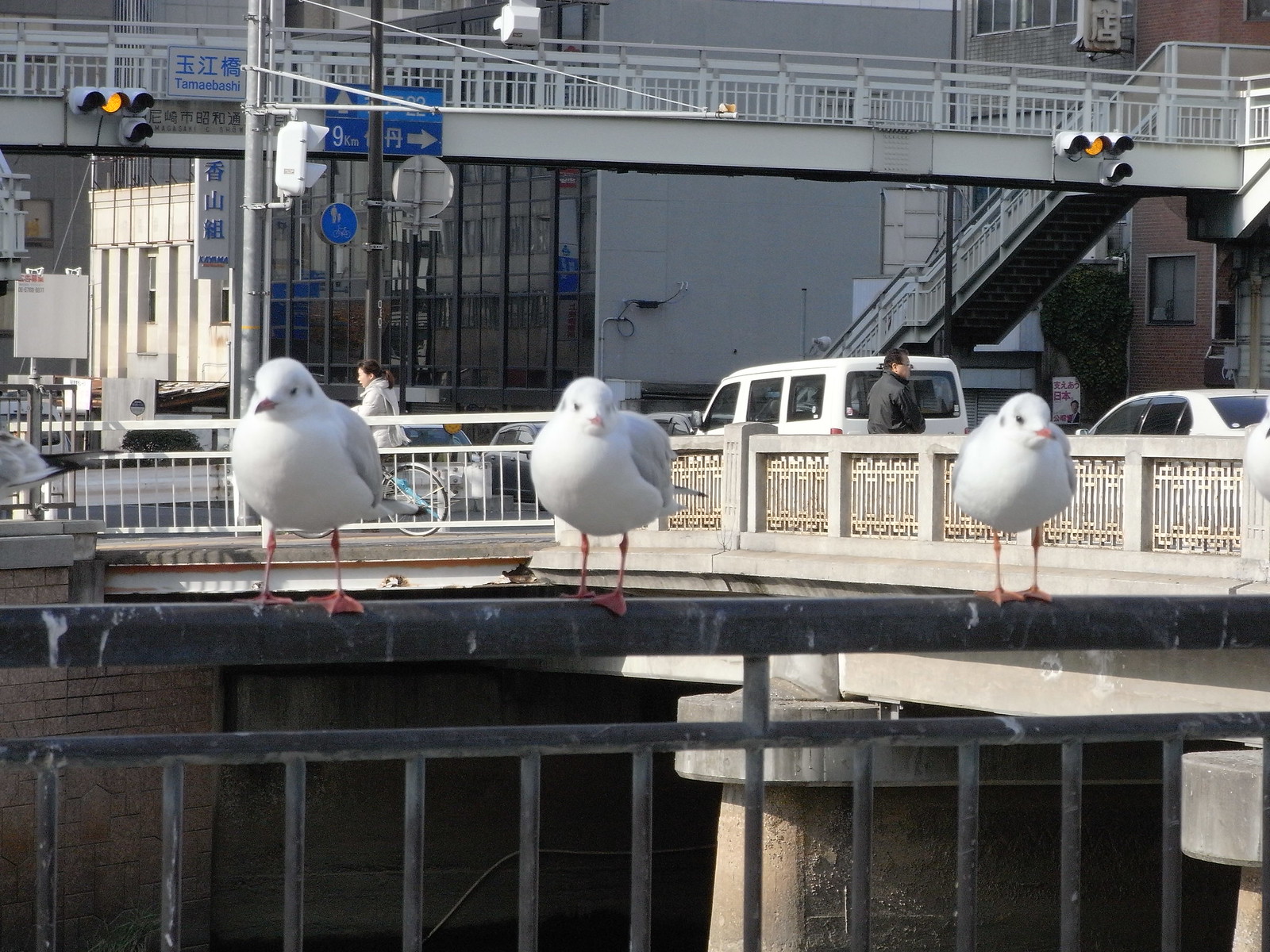The image captures three seagulls with orange webbed feet and a mix of white, grey, and black plumage perched on a black handrail in the foreground. This handrail borders a recessed area leading down to a waterway. To the right, a beige stone bridge spans the water. Across the water, a cyclist in a white jacket rides along a road where several cars are either stationary or merging into the traffic. The backdrop includes a white building with large glass windows and blue street signage featuring Japanese kanji characters, particularly "Tomei Bashi" in blue. The scene also contains a white handrail, a brick retaining wall, and a staircase ascending from the sidewalk to an elevated level. The overall setting likely depicts a bustling street in Japan, highlighted by the presence of distinct blue Chinese lettering signs and busy urban landscape elements, like traffic lights and commercial buildings.